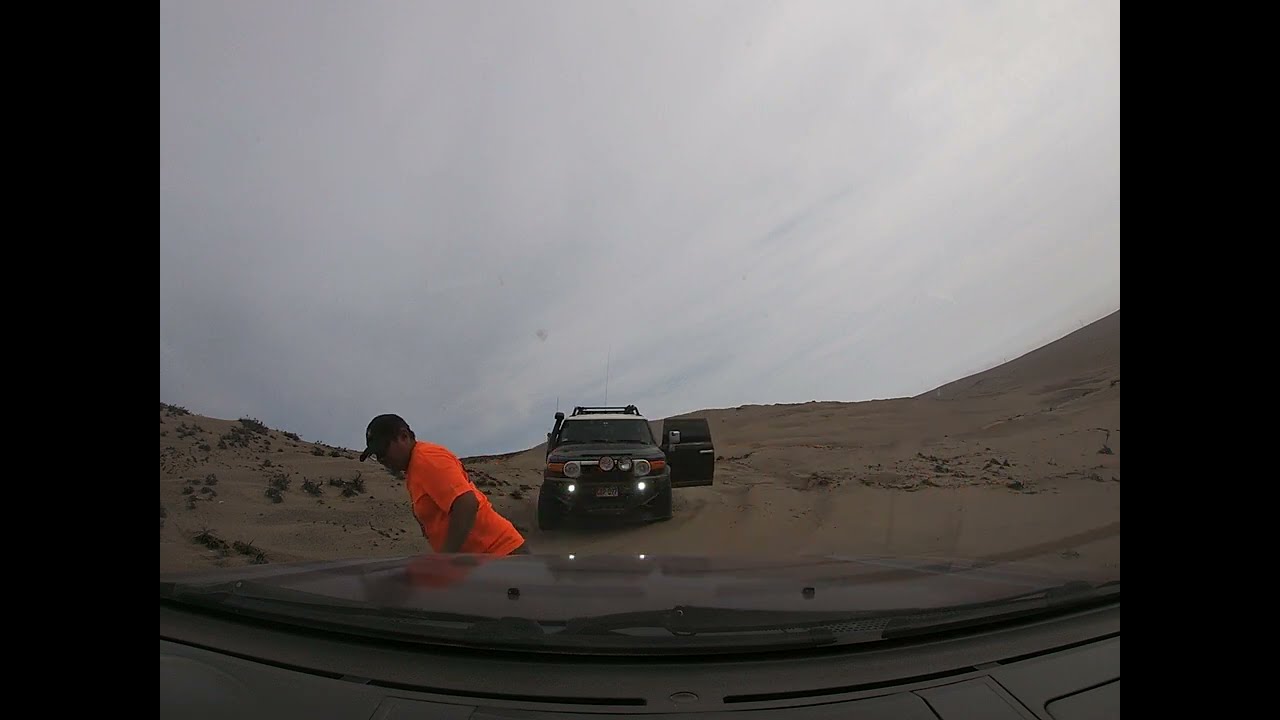The image is a color photograph taken from inside a parked vehicle, possibly through the dashboard window, capturing an outdoor desert setting. The road appears sandy with small patches of vegetation, giving the impression of dunes or elevated hills in the background. In the foreground, a man wearing a bright orange short-sleeved shirt and a dark hat bends over, seemingly examining the driver's side tire of the vehicle. Behind him, slightly to the right, stands a Land Rover-type vehicle with its fog lights on and the driver's side door open, suggesting it might be where the man exited from. The sky is an overcast gray, with only traces of blue visible, indicating an impending change in weather, likely rain. The overall atmosphere is dry and it seems to be late in the evening, just before dusk.